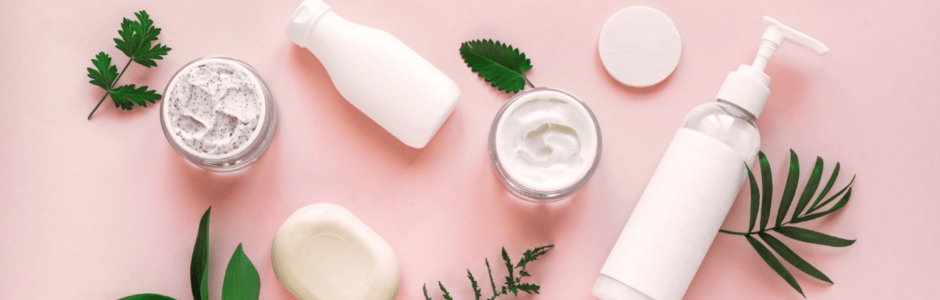This professional skincare advertisement showcases an array of beauty products on a vibrant pink background. The products, all in white containers, are meticulously arranged alongside green leaves, herbs, and plants, emphasizing their natural ingredients. From left to right, the layout includes a bar of ivory-toned soap at the bottom-left, flanked by two leaves. Above this is a glass jar containing exfoliating cream, identifiable by its white content speckled with deep purples and pinks. Adjacent is a white bottle with a flip cap. Centrally positioned is a small tub of cream, and to its right, a cotton cleansing pad. At the top-right is a diagonal bottle with a blank label and pump dispenser, likely for lotion. Scattered around these items are various sprigs, including miniature palm fronds and possibly parsley, enhancing the natural and organic theme of the products. Deep pink shadows cast by the items further contribute to the image’s stylized, appealing aesthetics.